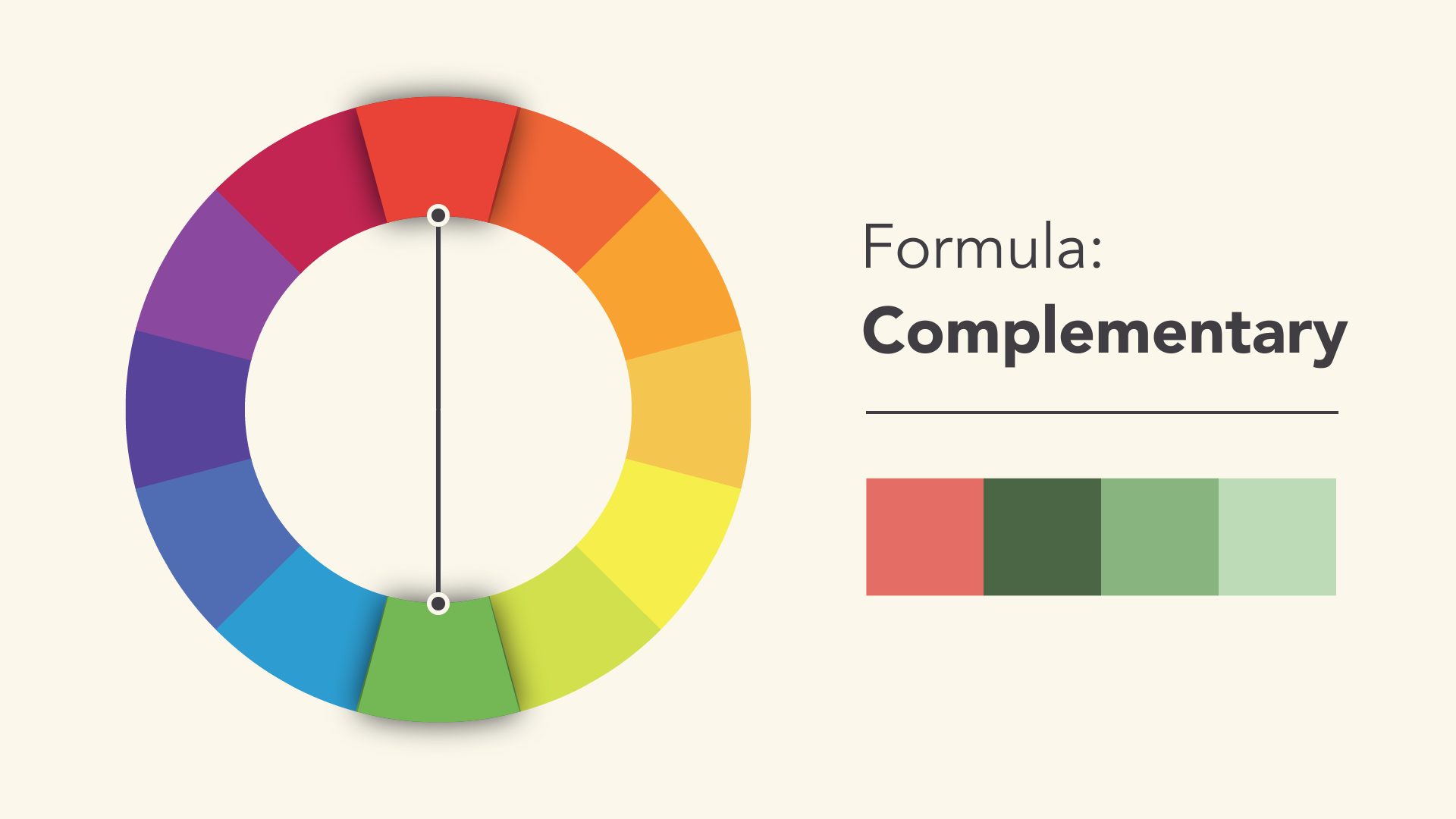The image presents a digitally created advertising chart with a beige or gray background. Dominating the left side is a color wheel featuring a gradient of hues arranged in a circular pattern: starting at the top with red, transitioning through shades of purple, blue, green at the bottom, turning yellow, orange, and returning to red. The circle is intersected by a thin black line connecting the top red and bottom green segments. 

On the right side of the image, the centerpiece of the chart is the text "Formula: Complimentary" in bold black letters. Below this text is a thin black line, followed by a horizontal bar composed of four color blocks arranged from left to right: reddish, dark green, lighter green, and very light green.

This detailed diagram effectively illustrates a full spectrum of colors, emphasizing both the cyclical nature of the color wheel and their complementary relationships, making it an informative visual for understanding color theory.